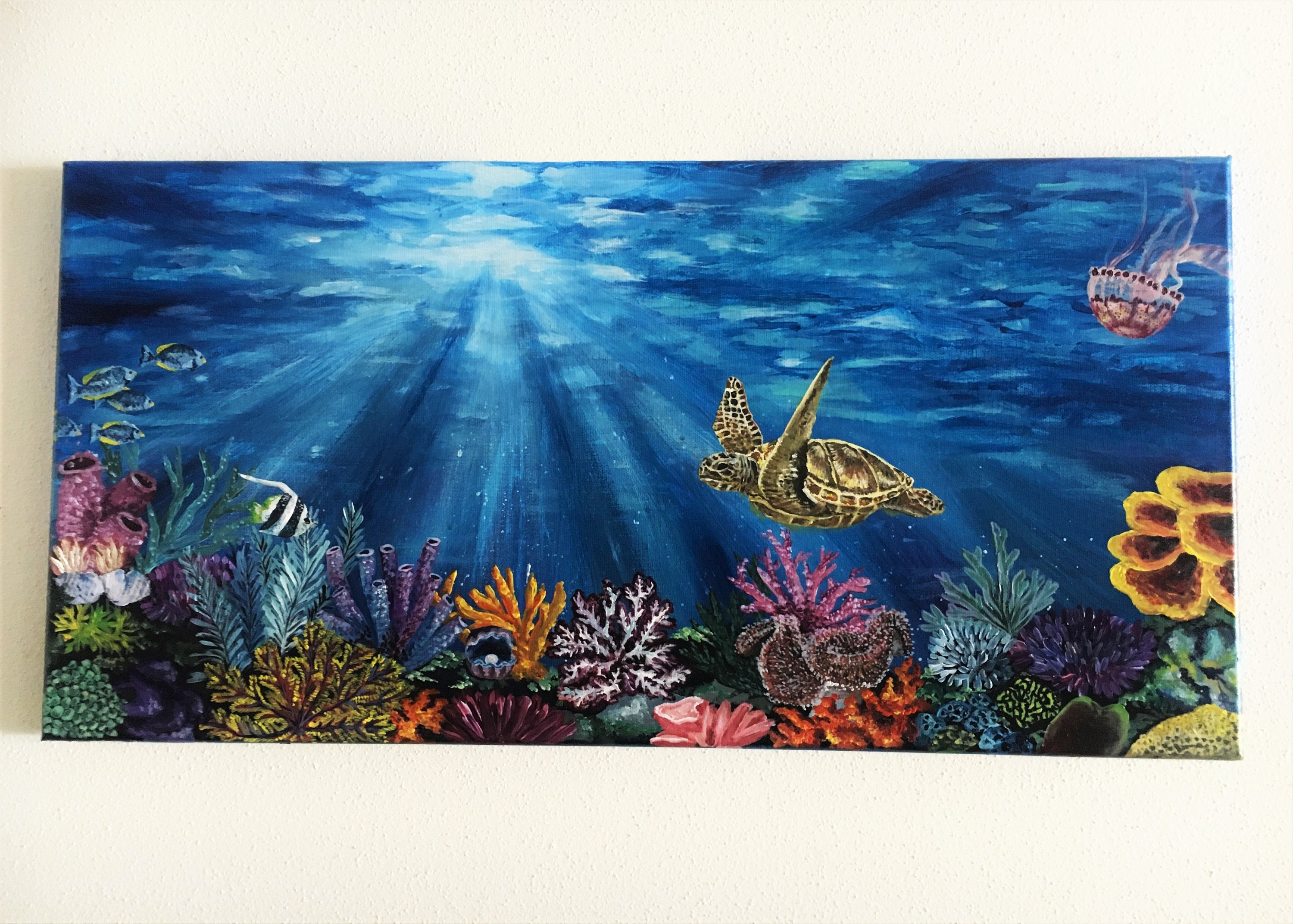This detailed painting presents an intricate underwater scene likely depicting marine life in the Pacific, possibly around the Galapagos Islands, against a plain white background. The canvas captures the essence of sunlight filtering through the water, illustrated with varied shades of blue and white, giving the effect of sun rays streaming down into the sea. Prominently featured in the middle is a large sea turtle, its flippers outstretched, showcasing a hard shell in hues of green, yellow, and brown. Surrounding the turtle, bright and colorful corals and sea plants in vibrant pink, orange, green, and yellow flourish at the bottom of the painting. To the left, a school of tropical fish swim, including zebra-striped fish in black and white, as well as others in vivid blue and yellow. In the upper right corner, a pink jellyfish, with delicate tentacles, drifts downwards. The detailed coral and flora create a vivid underwater tableau that brings to life the rich ecosystem of the ocean.